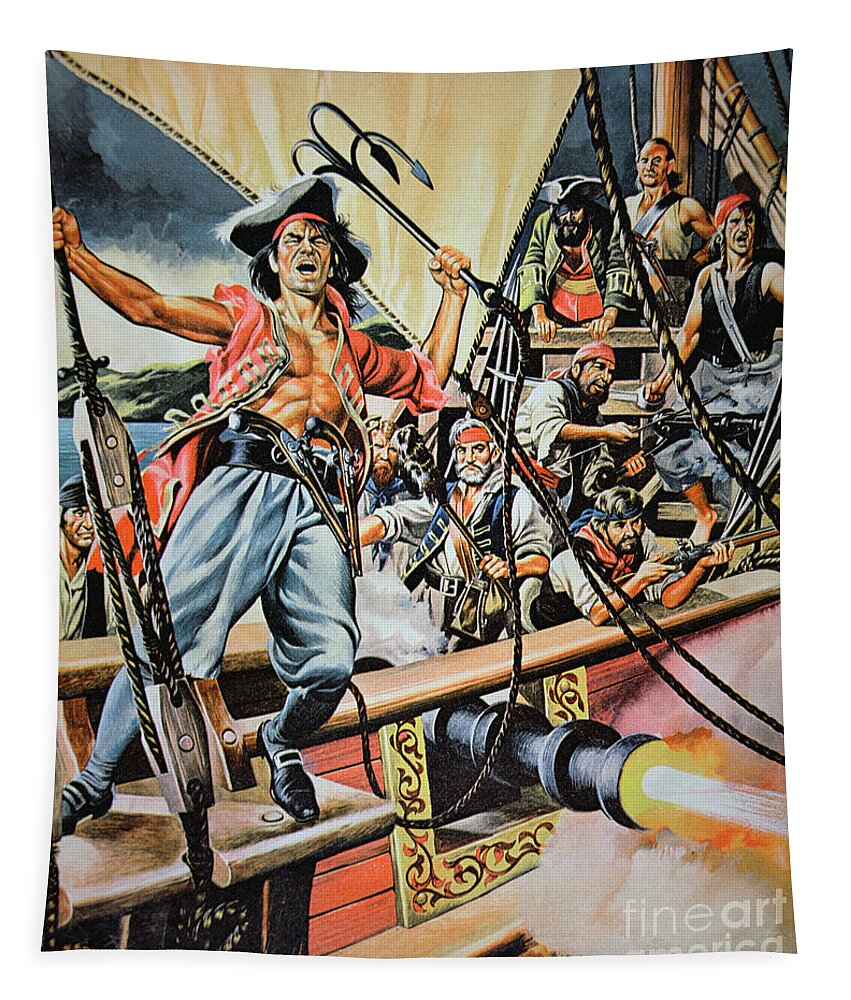This detailed painting by Fine Art America captures a dynamic scene aboard a pirate ship, employing a cartoony, comic book style. Central to the image is a bearded pirate with an open red shirt, billowy pants, and a thick belt adorned with large derringer-style pistols. This pirate is caught mid-action, about to throw a grappling hook from his left hand, seeming to aim at a nearby ship. Near him, members of his crew clad in various states of attire—ranging from red or blue bandanas to open shirts or vests—are actively engaging in the battle. A cannon fires prominently from the ship’s side, its muzzle flash illuminating the scene and adding to the sense of immediate danger. In the background, towards the bow, another figure wearing a captain's hat stands among approximately eight other pirates, contributing to the chaotic combat. The scene is rendered on a piece of cloth, which drapes imperfectly, giving the whole painting a tactile, handmade feel, and the words "Fine Art America" in white print mark the bottom right-hand corner.